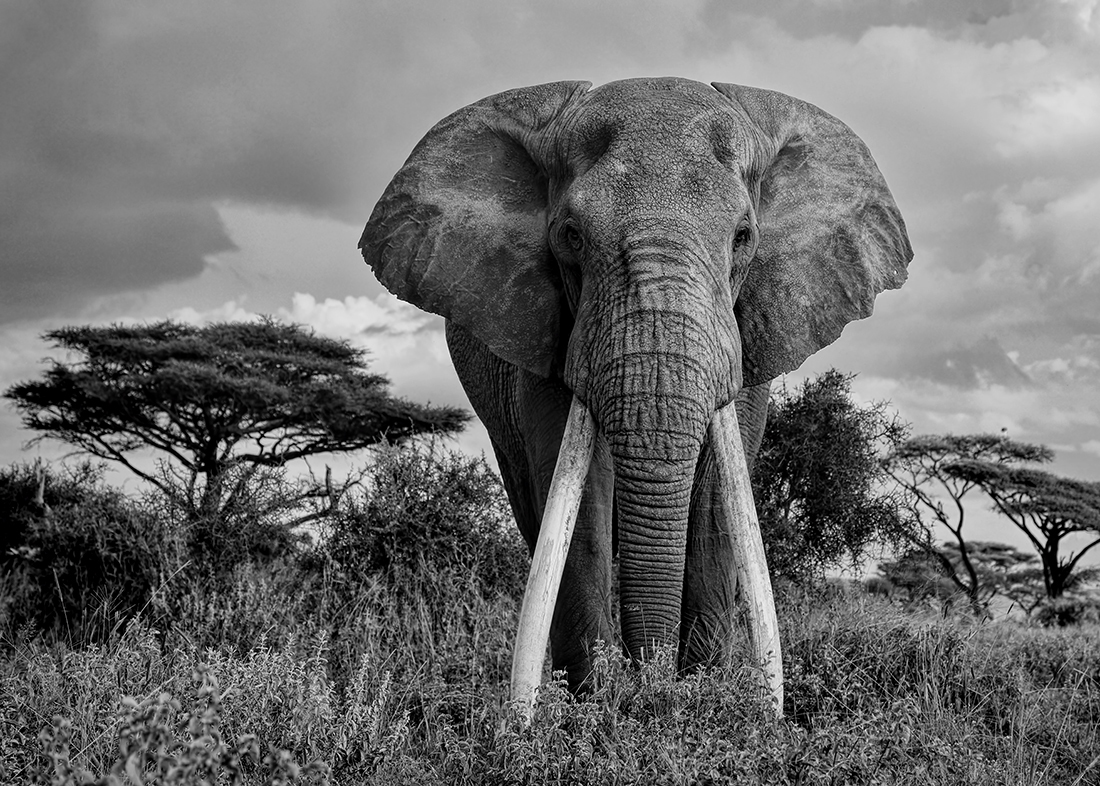This black and white photograph captures an imposing elephant standing in the African savannah. The elephant is slightly off-center, more towards the right, facing directly towards the viewer with its long tusks almost touching the tall grass that obscures its toes. Its large ears are down, and its legs are close together, creating a symmetrical and striking appearance. The thick foliage of the grassy field surrounds the elephant, leaving no bare ground visible. Medium-sized trees with wide, fanning branches rise on the left and right of the frame, marking the distant edge of the savannah. Above, the sky is a dramatic tableau of dark, gray clouds interspersed with some lighter, puffier ones, adding a sense of foreboding to the scene. The overall contrast in the image makes the elephant appear almost surreal, yet its presence commands attention, standing majestically in its natural habitat.